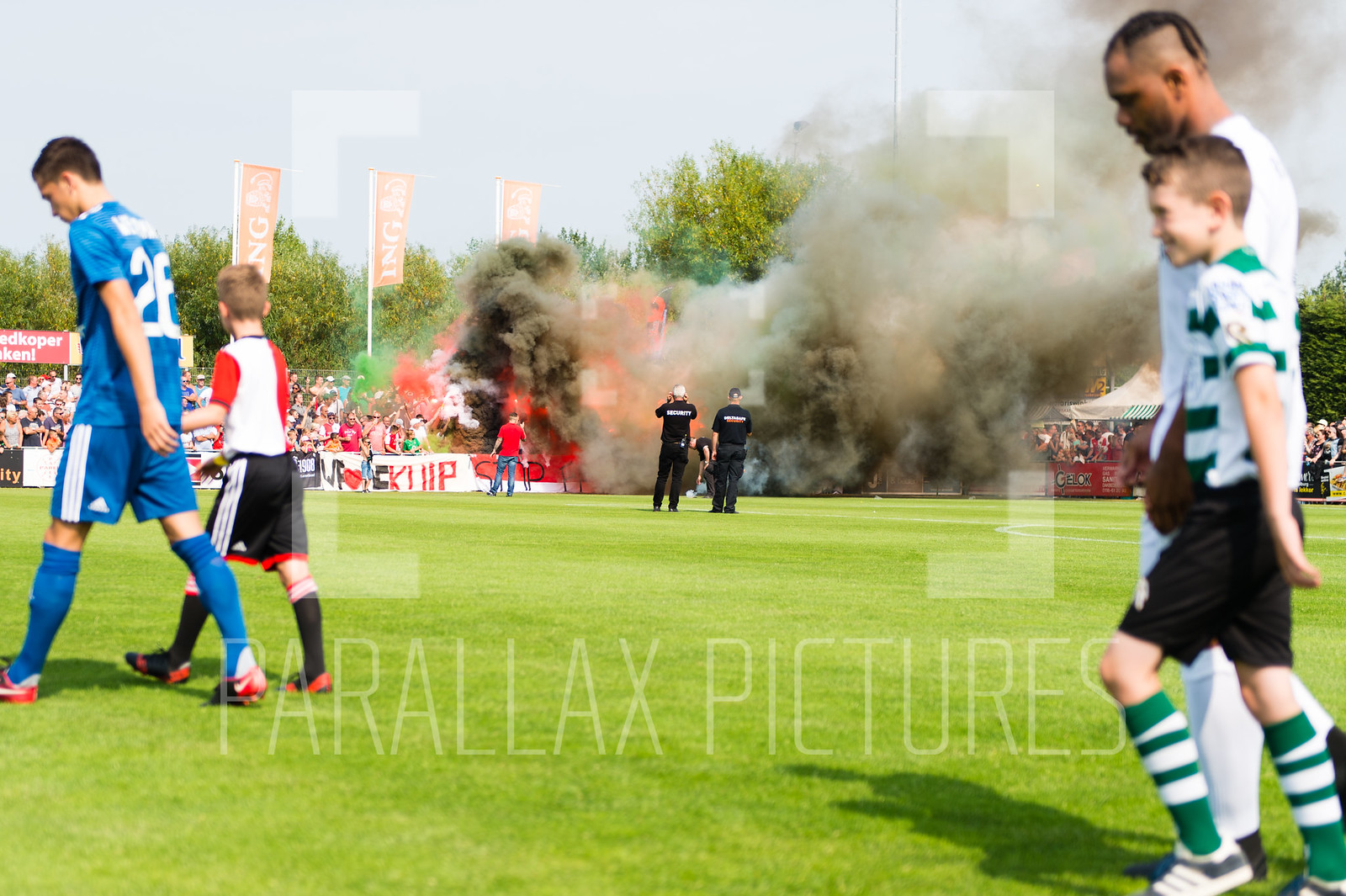In this full-color outdoor photograph, taken at a sporting event on what appears to be a pleasant summer day, we see a group of people on a lush green soccer field. The image captures two men and two boys, all dressed in different colored uniforms, likely indicating their involvement in the event. 

Leading the procession in the foreground, one man in a blue jersey is holding hands with a young boy in a red jersey, while another man in a white jersey holds hands with a boy in a green and white jersey. The backdrop of the photo includes an audience seated in the distance, calmly watching the scene unfold.

At the center of the image, two men in black t-shirts are recording what appears to be a fire or significant smoke, which, given the lack of concern from the crowd, seems to be intentional. There are visible flags fluttering, though the inscriptions on them are indiscernible. Adding to the detail, the photograph bears a watermark from Parallax Pictures.